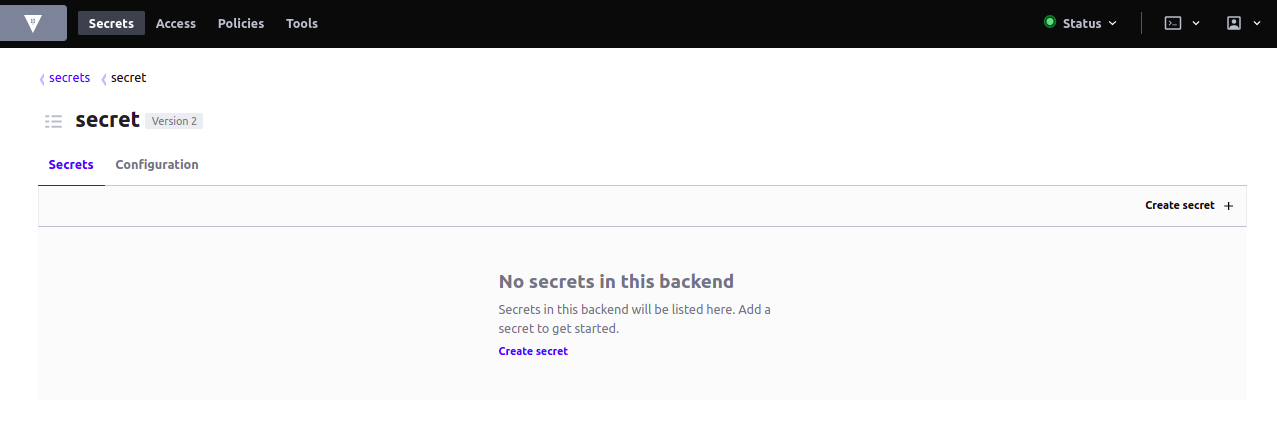The image is a screenshot of the top section of a website interface. The header features a prominent black banner. On the upper left side of this banner, there are several navigation tabs. These include, from left to right: a gray tab with an icon resembling an upside-down triangle, a "Secrets" tab, an "Access" tab, a "Policies" tab, and a "Tools" tab.

On the far right side of the banner, there is a "Status" tab, which includes a drop-down arrow indicating additional options when clicked. Next to it is another interactive tab, also featuring a drop-down arrow for further menu options. The final tab on the right is a profile square, which allows users to create an account and includes a drop-down arrow for extra profile-related options.

Beneath the black banner, on the left side of the screen, is some smaller text. The text "Secrets" is prominently displayed, followed by the subtext "Secret." Adjacent to this is a faint word that is unclear. Below the bold "Secret" text, it reads "Secrets Confirmation."

In the main body of the screen, there is a central message stating, "No Secrets in this back end."